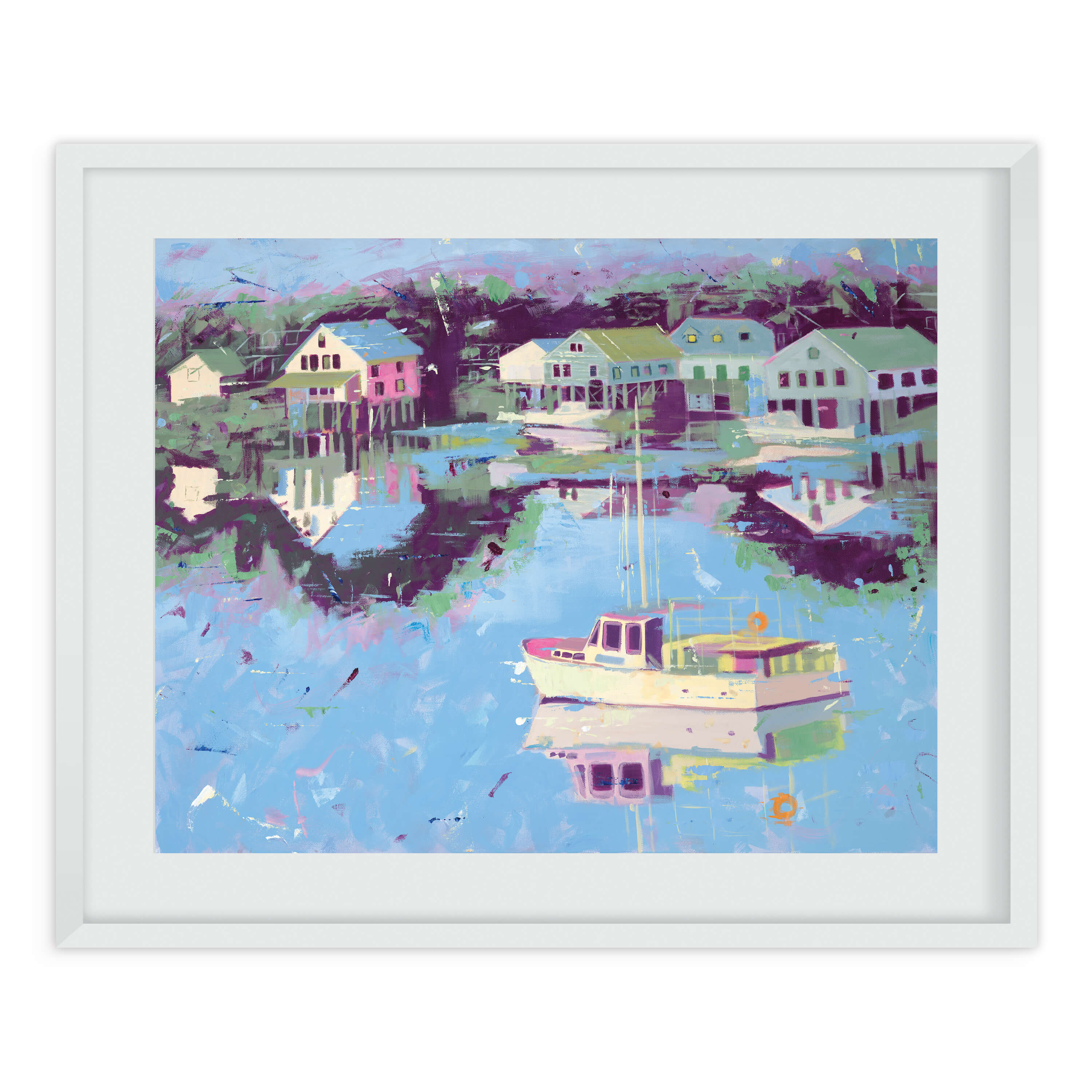This image is a beautifully detailed painting, likely created with traditional or digital art techniques. It features a serene ocean setting rendered in pastel tones. A boat is gracefully floating on the calm waters, providing a focal point in the scene. The background showcases quaint houses, adding a touch of human presence to the tranquil environment. The painting is framed with a light blue-gray border, complementing the overall color scheme and enhancing its presentation. The palette includes a soothing blend of green, white, purple, blue, black, red, and pink, bringing the scene to life with a harmonious mix of colors. This artwork is a captivating and vibrant portrayal of a peaceful coastal landscape, devoid of any text elements.